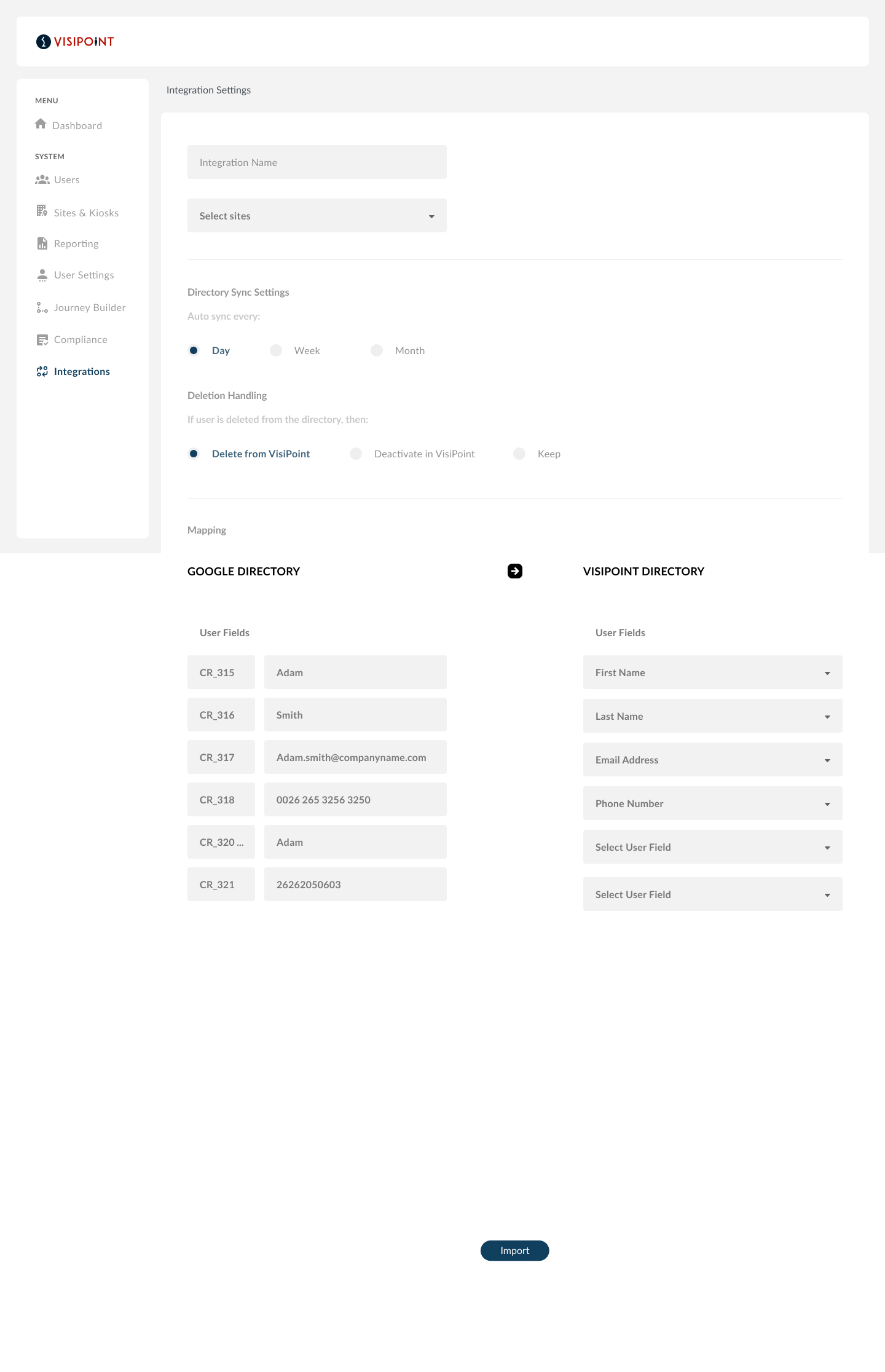**Detailed Caption:**

The image appears to be a screenshot of a mobile application interface with a predominantly white background and gray outlines around various sections. On the left side of the screen, there is a vertical dark gray menu featuring a list of sections: 

1. Dashboard
2. System
3. Users
4. Size and Links (possibly "Sinks")
5. Reportings
6. User Settings
7. Journey Builder
8. Compliance
9. Integrations (highlighted in blue)

On the right side of the screen, the focus is on the "Integration Settings" section. Below this title, the interface displays options for "Integration Name" and "Select Sites," which likely includes a dropdown menu. 

Further down, there are "Directory Sync Settings" with three selectable synchronization frequencies: day, week, or month, and the day option is currently selected. 

Further options include "Destination Handling" with "Delete from Visit Point" selected. Below this, there is a "Mapping" section that appears to link a Google directory. This directory contains various entries listed under names. To the right, there is a "Visit Point Directory" with user fields, indicating some form of structured data applicable for either user management or system integration purposes. 

The overall interface suggests it is a technical tool, possibly for managing system integrations, directory synchronization, and user data mapping.